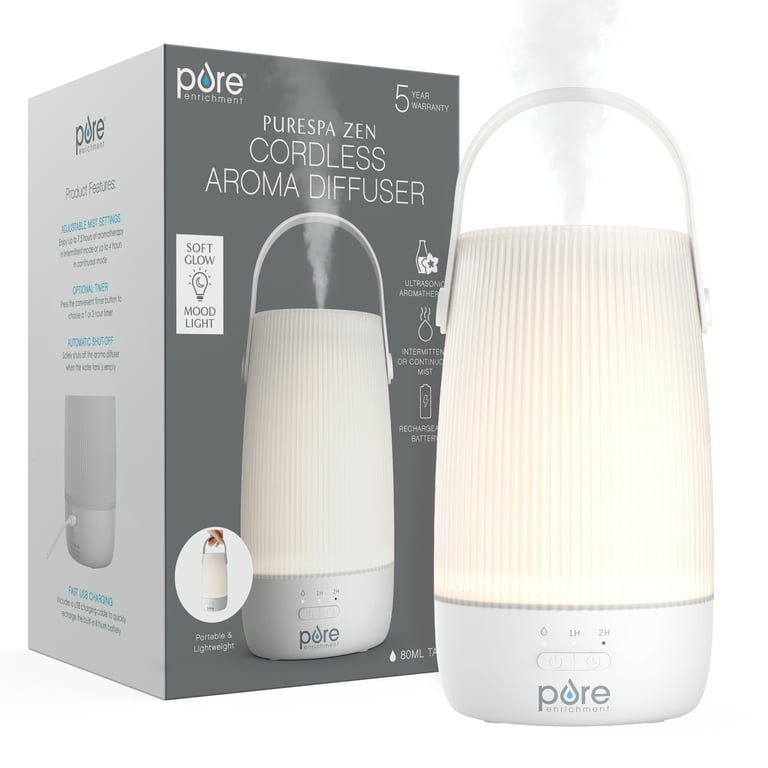This image features a cordless aroma diffuser from Pure Enrichment, displayed alongside its box against a white background. The sleek, all-white diffuser includes a white handle on the top and a white plastic base. It proudly bears the "Pure Enrichment" branding and is equipped with two buttons on the front: one marked with a water droplet, labeled "1H," and another marked "2H."

The packaging is detailed and informative, showcasing a gray front panel that displays the diffuser with the words "PureSpa Zen" and "Cordless Aroma Diffuser" in white text. The top left corner highlights the "Pure" logo, featuring a raindrop design in the 'O' with blue coloring. The top right corner denotes a 5-year warranty. The side of the box, also gray, lists the product's features in white text. A white panel on the box includes the phrases "Soft Glow Mood Light" and a light bulb icon, with gray and blue lettering. At the bottom of the packaging, "80ml" is noted alongside a white raindrop icon, indicating the diffuser's capacity. The product's description on the box encompasses a variety of fonts and colors, blending blue, gray, and white to emphasize its functionalities and aesthetics.

The side panel of the box reveals more features, starting with the word "Product features," but the exact text remains partially unreadable due to the angle. The actual diffuser, positioned to the right of the box, mirrors the box's design ethos, boasting a clean and minimalist appearance that complements its functional attributes.